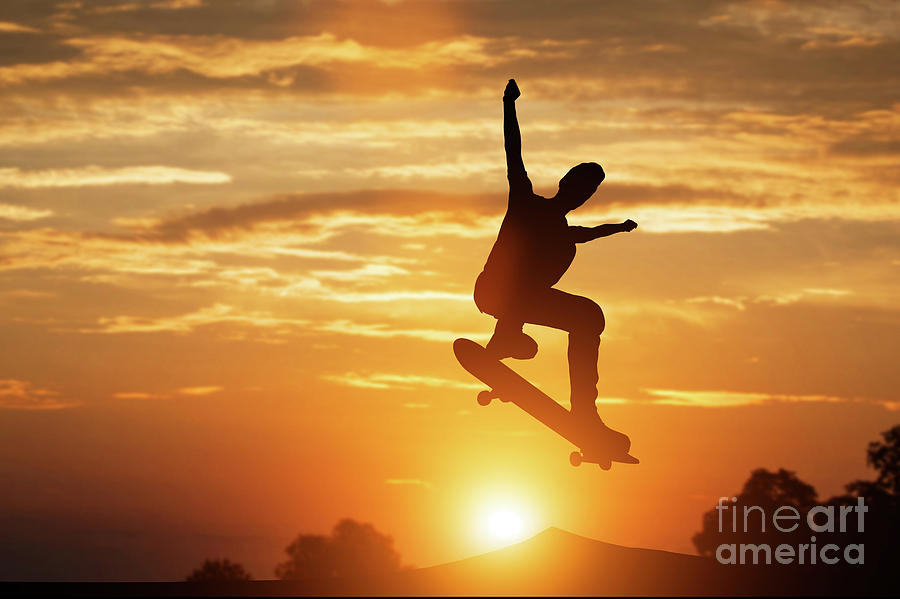In this striking photograph by Fine Art America, the sky is ablaze with the vibrant hues of a sunset, ranging from deep oranges to soft grays. The sun, low on the horizon, casts a mesmerizing glow that illuminates a few scattered clouds and silhouettes a distant landscape that includes a hill and three distinct trees. At the center of this vivid scene, a skateboarder is captured mid-air, arms raised high. The figure and the skateboard are rendered entirely in shadow, with no discernible features, emphasizing their dynamic pose against the brilliant backdrop. The skateboarder’s silhouette even reveals spiked hair, adding to the sense of motion. Below the skateboarder, the hill forms a perfect base for the sun’s ascent, framing the scene beautifully and making it an iconic moment of action and natural beauty.